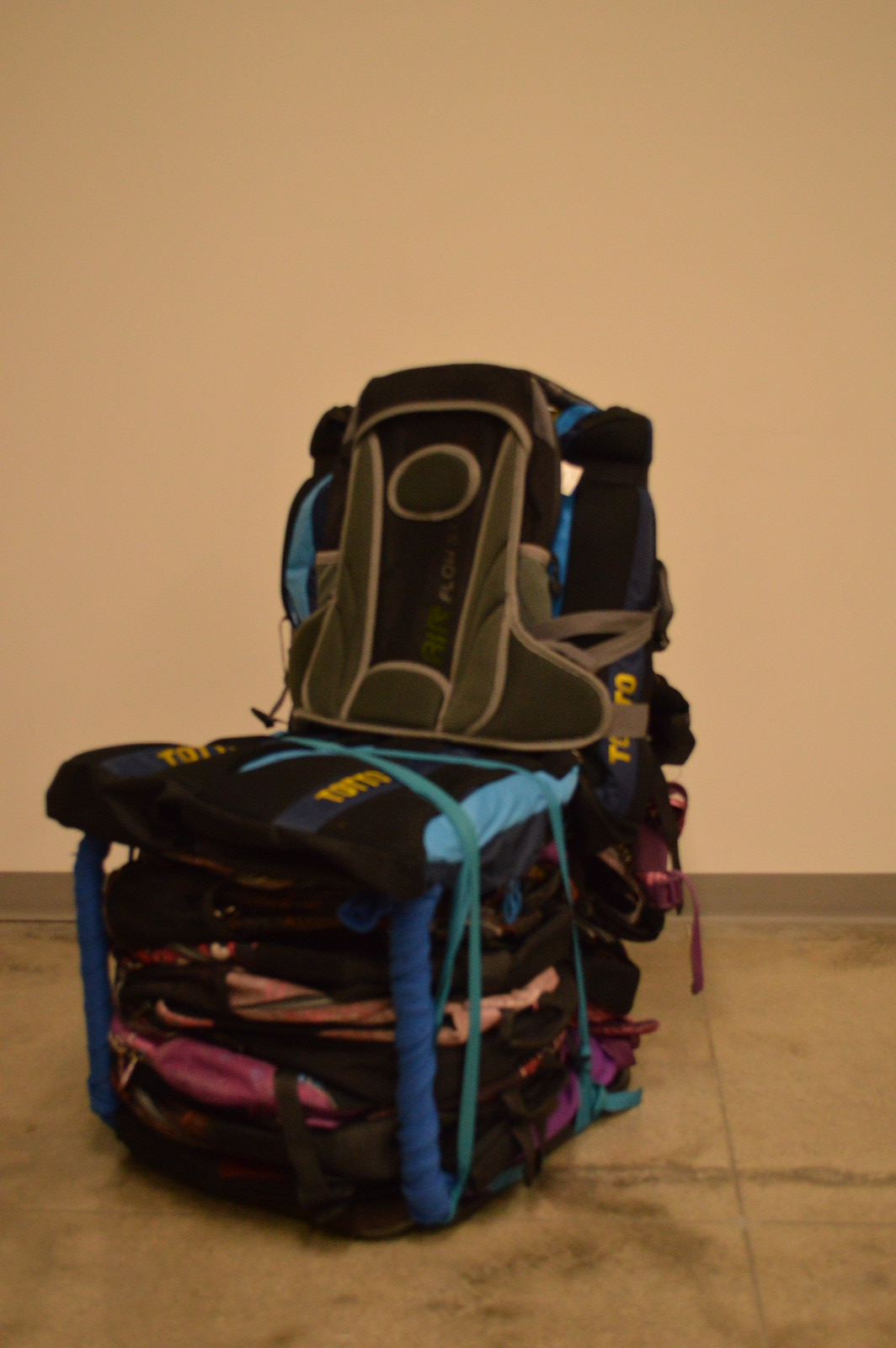This is an amateur photo depicting a makeshift chair crafted from flattened and stacked backpacks, primarily blue and black with splashes of pink. The main part of the chair appears to be constructed from seven different backpacks, crisscrossed and tied together with turquoise blue bungee cords. The backrest consists of an additional three to five backpacks, meticulously laced to form a seatback. The seat backs and some gray padding are stacked underneath, providing additional support. The background features an eggshell white wall, complemented by brown flooring with a gray vinyl baseboard. Notably, the letters "TOTO" are written in yellow on multiple sections of the chair. The overall scene is bathed in yellowish lighting and portrays a creative, makeshift seating solution, possibly intended for temporary use, such as camping. There is no text or date stamp to provide further context.